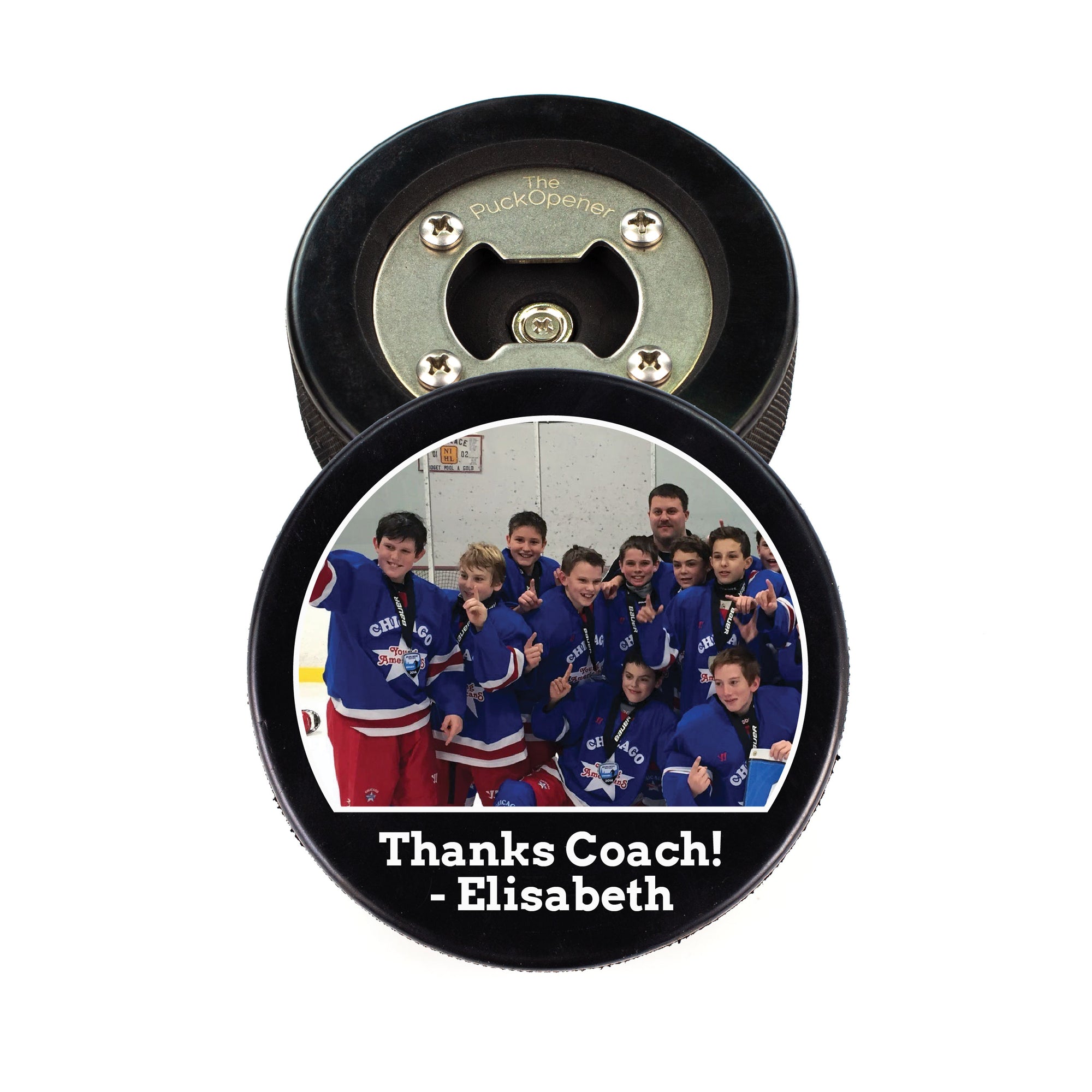Detailed Caption: The image features a unique hockey puck that has been cleverly designed to function as a bottle opener. The puck itself appears to be a standard black hockey puck, but the top can be removed to reveal the bottle opening mechanism inside. The method of removing the top could be by popping it off or unscrewing it, though the specific mechanism isn't clear as threads are not visible on the main body of the puck.

Upon opening the puck, the interior reveals a metal bottle opener inset, characterized by a shape resembling a dog bone—wider at the ends and narrower in the middle—crafted to fit over the cap of a bottle and facilitate easy opening. Engraved into the metal is the branding "The Puck Opener."

The detached top of the puck features a vibrant group photo of a children's hockey team. The young players are clad in blue jerseys that prominently display "Chicago" in white lettering. Centered below the word is a white star adorned with a blue and red icon, bordered by a band. Their jerseys are further accented with white and red trim at the bottom and a band on the arm. Complementing their jerseys, the team dons red shorts. They stand proudly on the ice within an arena, with a light-colored background and floor, marked by a distinguishing yellow warning line at the base of the wall.

Adding a personal touch to this keepsake, the bottom portion of the image contains a heartfelt inscription in white letters, reading: "Thanks, Coach Elizabeth." This detail transforms the functional item into a cherished memento.